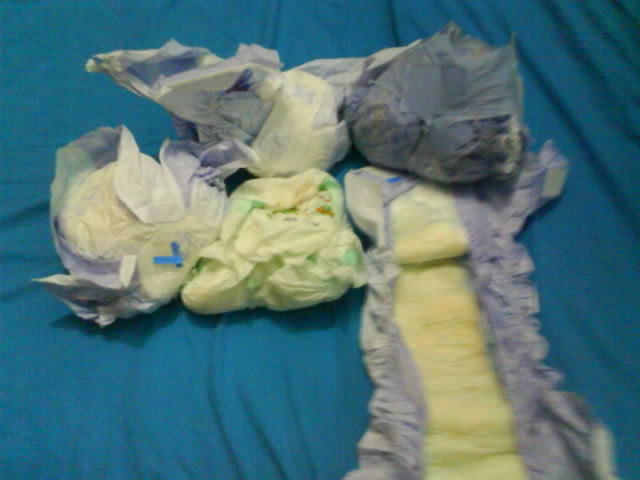The image is a close-up view of a blue fabric, possibly a wrinkled towel or sheet. On this blue background, there are several disposable diapers, most of which appear to be soiled and neatly rolled into balls. The colors of these diapers vary: some are predominantly purple with white in the middle, others are cream-colored with green designs, and there is a notably yellow one with green paper inside. In the lower right section, a heavily soiled diaper lies unfurled, showing a yellowish center. The image, though not very crisp, clearly suggests that these objects are diapers, with visible plastic strips securing the rolled ones and giving a sense of untidiness over the blue fabric.